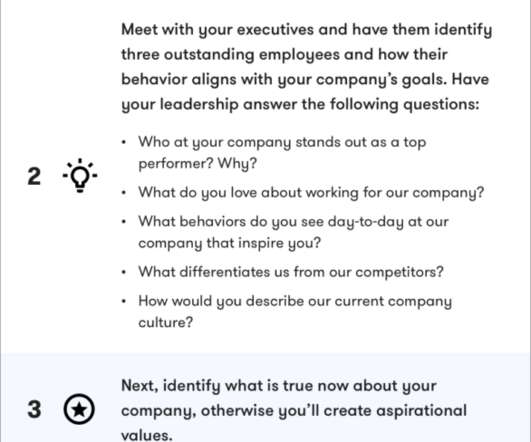Screenshot of a Website: Detailed Steps for Leadership Evaluation

This screenshot captures a structured guide aimed at company executives for employee evaluation and company culture assessment. The visual presentation features thin vertical lines on both the left and right margins, adding a clean framing to the content. Midway down the image, a bold numeral "2" is prominently displayed, accompanied by a light bulb icon, signifying an important step or idea.

At the top, in bold black text, the instruction reads: "Meet with your executives and have them identify three outstanding employees and how their behavior aligns with your company's goals. Have your leadership answer the following questions:" This introduction sets a clear directive for the executive meeting.

Below this, in lighter, finer print, a series of bullet points enumerate the specific questions to be addressed:
- Who at your company stands out as a top performer? Why?
- What do you love about working for your company?
- What behaviors do you see day to day at our company that inspire you?
- What differentiates us from our competitors?
- How would you describe our current company culture?

Near the bottom, the numeral "3" appears in bold with a distinctive circle enclosing a star, drawing attention to the subsequent step. This section states in bold print: "Next, identify what is true now about your company, otherwise you'll create aspirational values." It is highlighted with a light gray background, emphasizing the critical nature of aligning current realities with company values to prevent creating merely aspirational, rather than practical, goals.

This detailed visual guide serves as a comprehensive tool for leadership to reflect on and enhance employee performance and company culture.